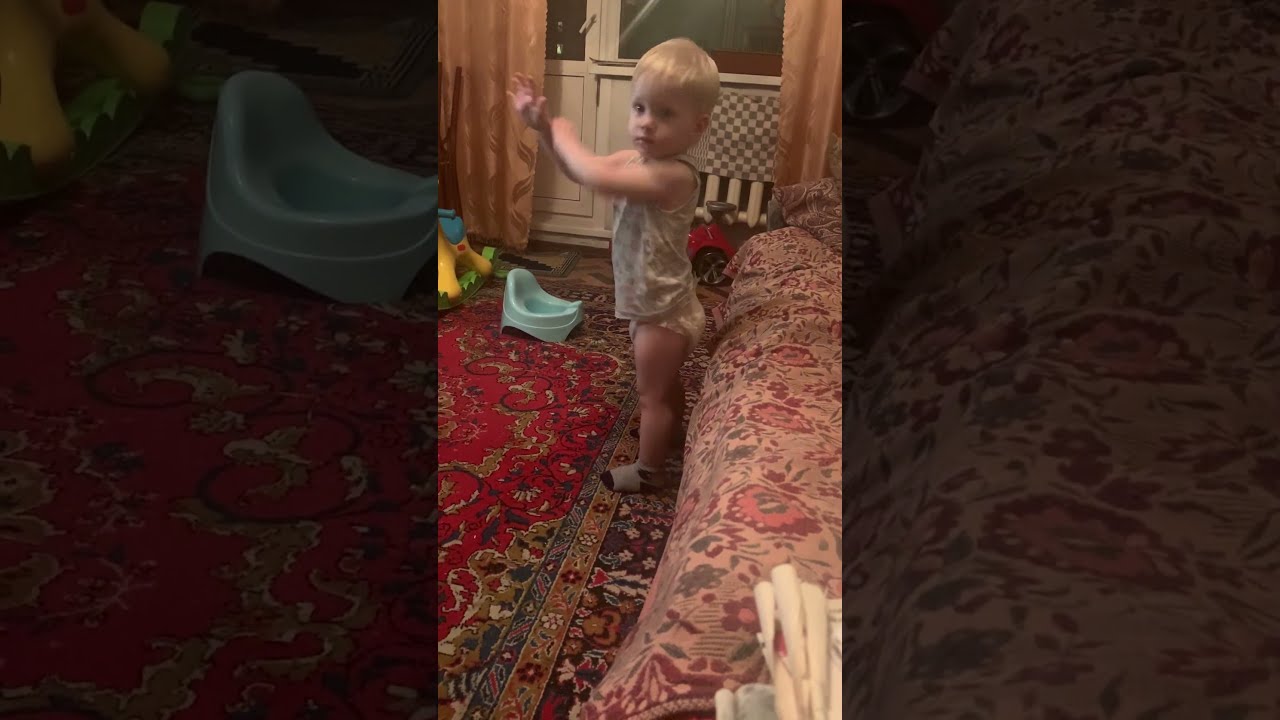This indoor photo captures a lively scene featuring a little toddler with short, very light blonde hair, who is standing up with their arms raised, seemingly trying to get the attention of an adult. The toddler, whose gender is not clearly identifiable, is dressed in a tank top, diapers, and socks. They are positioned in the center of a warmly colored living room, standing on a very ornate and colorful rug dominated by shades of red, with intricate floral patterns that also incorporate touches of dark red, beige, blue, white, and browns. Surrounding the child, there's a vibrant, flower-patterned blanket or throw on a bed or sofa, adding to the room's colorful decor. In the background, you can spot beige-colored drapes that contrast with the pink curtains on the window. Additionally, a blue training potty is placed nearby. Various toys are scattered on the floor, suggesting an active playtime. A door and a sofa are visible in the room, framing this cozy and dynamic family scene.